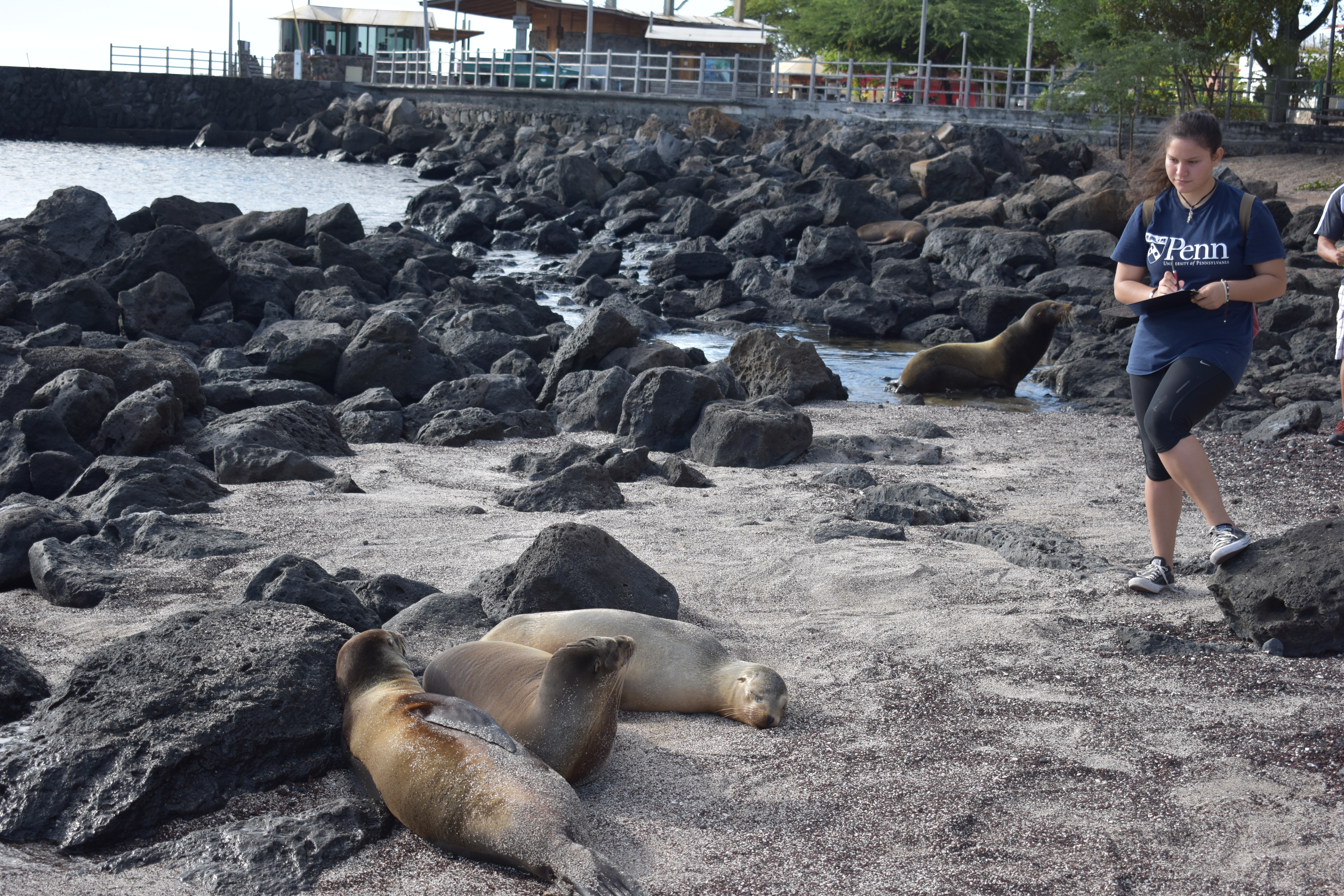In this captivating photograph, we find ourselves on a rocky beach, possibly situated in Southern California, given the presence of seals comfortably lounging around. The shoreline is composed of dark, volcanic-looking rocks and a stretch of gray gravelly sand, which creates a stark contrast with the light brown hues of the seals. 

In the foreground, a young woman, who appears to be in her late teens, is standing, partially leaning on one of the black rocks. She is dressed in a navy blue "Penn" t-shirt from the University of Pennsylvania, black shorts, and track shoes. She holds a notepad in her hand, suggesting she might be documenting the scene, possibly as a student or researcher.

On the bottom left of the frame, there are three seals resting on the gravelly sand, with one of them glancing up at the young woman while the others seem to be asleep. To her right, yet another seal is emerging from the water, joining the others on the beach. 

In the background, there is a pier with a small building at its base, and green trees can be seen further back, providing a lush frame to the scene. The combination of the dark rocks, gray sand, and the serene assembly of seals, along with the focused young woman, creates an intriguing and picturesque coastal snapshot.